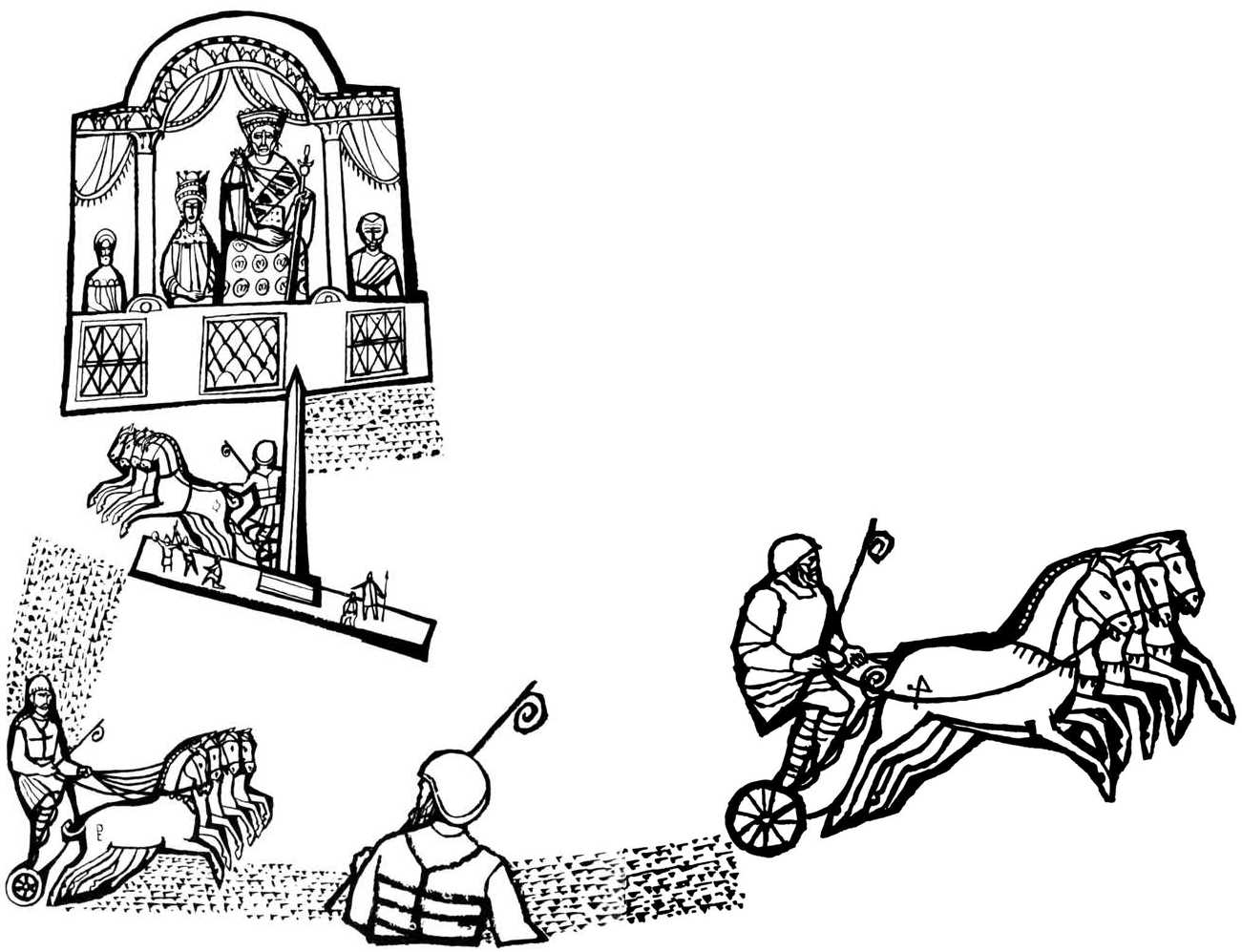This intricate black and white artwork captures various scenes of Roman or medieval life. At the top left, a regal viewing area with pillars and curtains showcases a king holding a scepter and a queen beside him, both observing the events below. The royal entourage, including other nobles, stands nearby. Below them, the scene transitions to a lively arena where a chariot race unfolds. On the bottom left, a man in a chariot pulled by four horses charges forward, matched on the right by another charioteer, similarly equipped with four horses and a helmet, gripping the reins tightly. Centered in the piece, a helmeted figure holding a lance oversees the dirt path that cuts through the illustration. The detailed portrayal, reminiscent of scenes that might appear in a medieval or Roman-themed coloring book, beautifully captures the essence of historical grandeur and the thrilling spectacle of chariot racing.